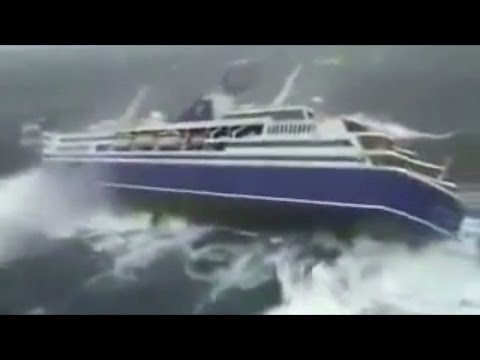In this detailed drawing, a massive ship braves a tumultuous sea under a foreboding, dark gray sky. The ship, with a blue and black hull and a white superstructure, features numerous windows and a prominent, black captain's window at the top. It's angled precariously to the back right of the image, suggesting it might tip over due to the rough waves. The ocean below is a dark greenish-blue, frothing with white, choppy waves that crash against the vessel's sides. The stormy atmosphere is heightened by thick, black line segments framing the top and bottom of the image, adding a sense of encroaching doom. Despite the tempest, the ship, possibly a cruise liner or a large yacht, struggles to stay afloat, evoking feelings of peril and tenacity.